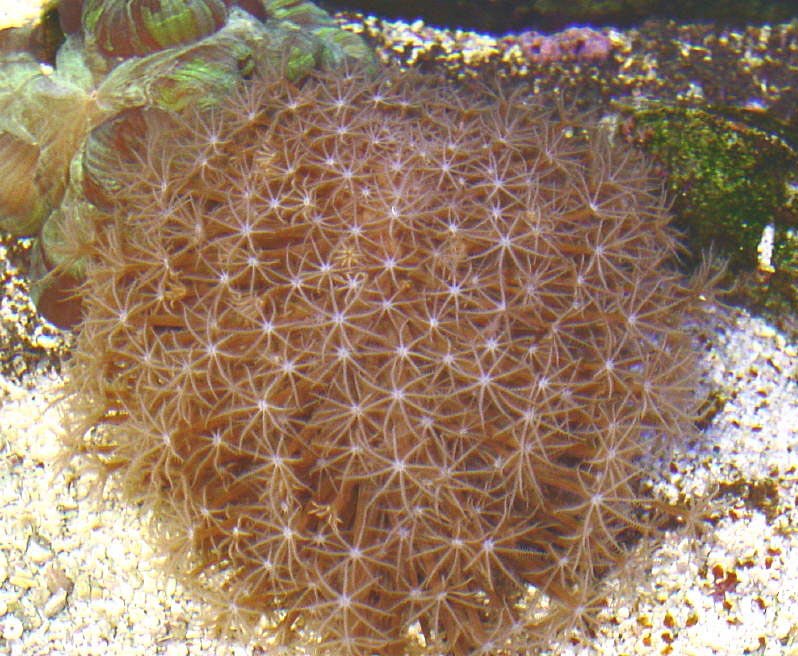This photograph most likely captures an underwater scene featuring a central brown object that resembles an intricate assembly of tangled strings. These strings converge to form a star-shaped pattern, reminiscent of a sea creature or plant. The object is adorned with numerous small, white, star-like formations, each with six protruding legs, giving it a distinctive, almost starfish-like appearance. This centerpiece is set against a backdrop of diverse greenery, including vibrant plants and moss-covered rocks, accentuated by bright purple and white flowers. The foreground consists of a bed of white gravel or sand, adding texture and depth to the image. The composition suggests a close-up, detailed view, focusing on the unique and almost ethereal qualities of the central object within its lush, underwater environment.